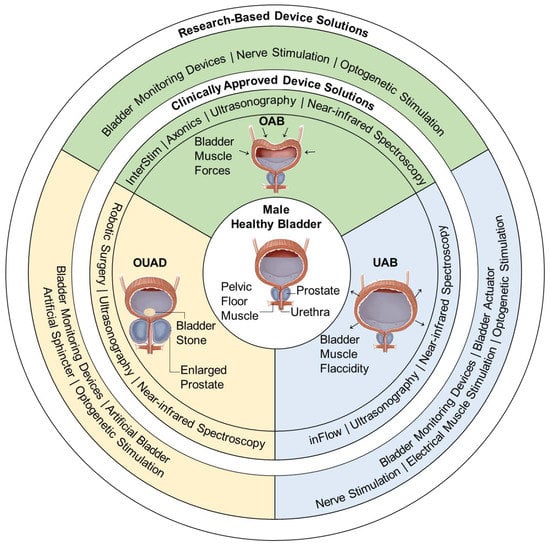The diagram is a detailed circular infographic focused on the male bladder and associated medical conditions and solutions. At its core, a central white circle is labeled "Male Healthy Bladder," illustrating key anatomical features such as the prostate, urethra, and pelvic floor muscle. Surrounding this central depiction is a secondary white circle labeled "Clinically Approved Device Solutions," which details various interventions, including bladder monitoring devices, nerve stimulation, electrical muscle stimulation, artificial bladder and sphincter, and optogenic stimulation. Outside this, a tertiary circle is labeled "Research-based Device Solutions," highlighting advanced technologies like robotic surgery, ultrasonography, near-infrared spectrography, and inflow. The diagram uses a color-coded system to visualize different conditions, such as bladder muscle flaccidity, enlarged prostate, and bladder stones, along with their respective treatment options, including Axonics and bladder actuator solutions. This concentric layout effectively communicates both the anatomy of a healthy male bladder and the spectrum of available diagnostic and therapeutic devices.